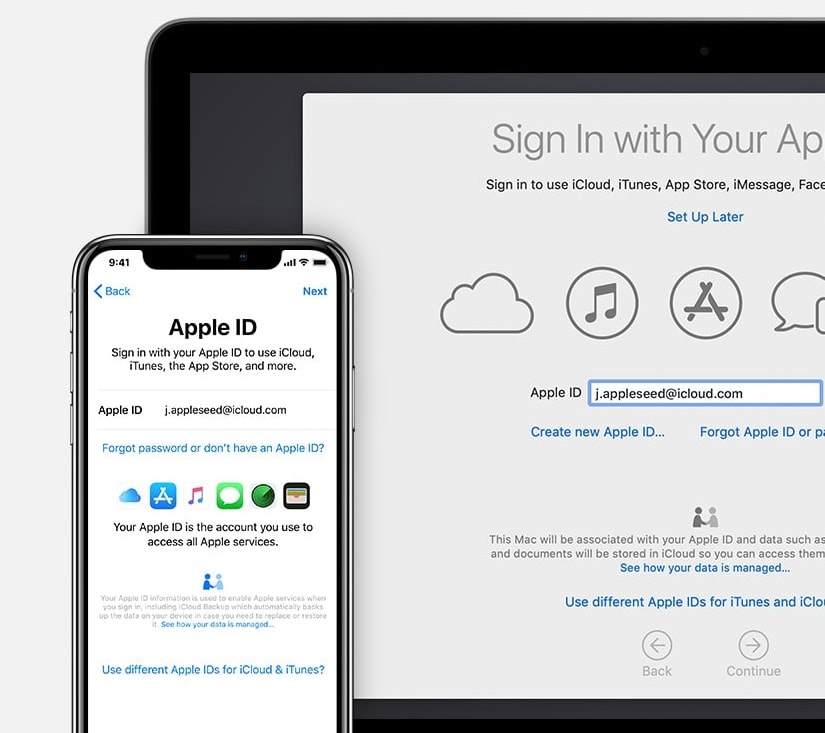The image depicts a screenshot showcasing both a tablet and a smartphone displaying an Apple ID sign-in page. On the tablet, a website banner reads "Sign in with your Apple ID," inviting users to log in to access services such as iCloud, iTunes, the App Store, iMessage, and Facebook. The text is presented in black on a white background, ensuring clarity and readability. Beneath this prompt, a blue hyperlink states "Set up later." Various service icons are visible, including the iCloud symbol, iTunes' musical notes, the App Store's stylized "A," and iMessage's speech bubble icon. The Apple ID input box is pre-filled with "jAppleSeed.icloud.com."

The smartphone displays a similar layout, adapted for a mobile interface. It includes an input box where users can sign in with their Apple ID. Below the input area are links for "Create new Apple ID" and "Forgot Apple ID," provided in footer text. The mobile version maintains the same visual elements and functionalities as depicted on the tablet, ensuring consistency across devices.